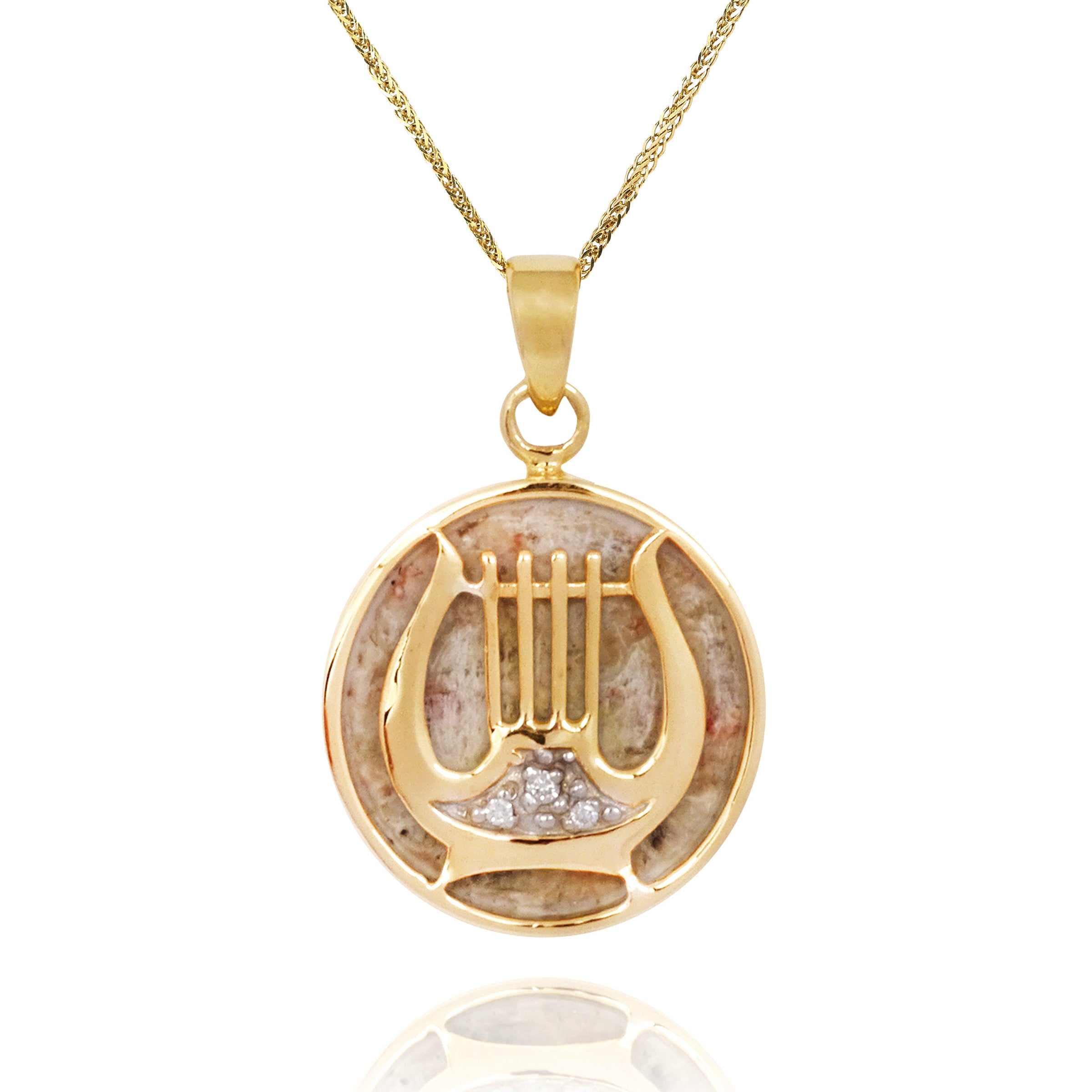This is a detailed photograph of a vintage gold pendant, elegantly suspended from a thin gold chain with a prominent chain ring securing the attachment. The pendant is circular in shape with a raised, intricate harp design that evokes the whimsical image of a fantasy creature’s harp, rather than a traditional orchestral one. The harp is outlined in shiny gold and features a central section embellished with what appears to be diamonds or cubic zirconia, adding a touch of sparkle.

The surface of the pendant’s face resembles a marble-like material, tinged with a pink hue and adorned with subtle, intricate textures. This background gives it an old-world charm reminiscent of ancient Roman jewelry, further enhanced by suggestions of floral fabric designs or opalescent colors like maroon, gray, and white.

Set against a solid white background that reflects part of the pendant, the entire composition underscores the pendant’s aged elegance and the fine craftsmanship that has gone into its creation. The golden elements, including the chain and harp design, remain highly polished and radiant, contrasting with the pendant’s textured backdrop, giving it a timeless yet eye-catching appeal.